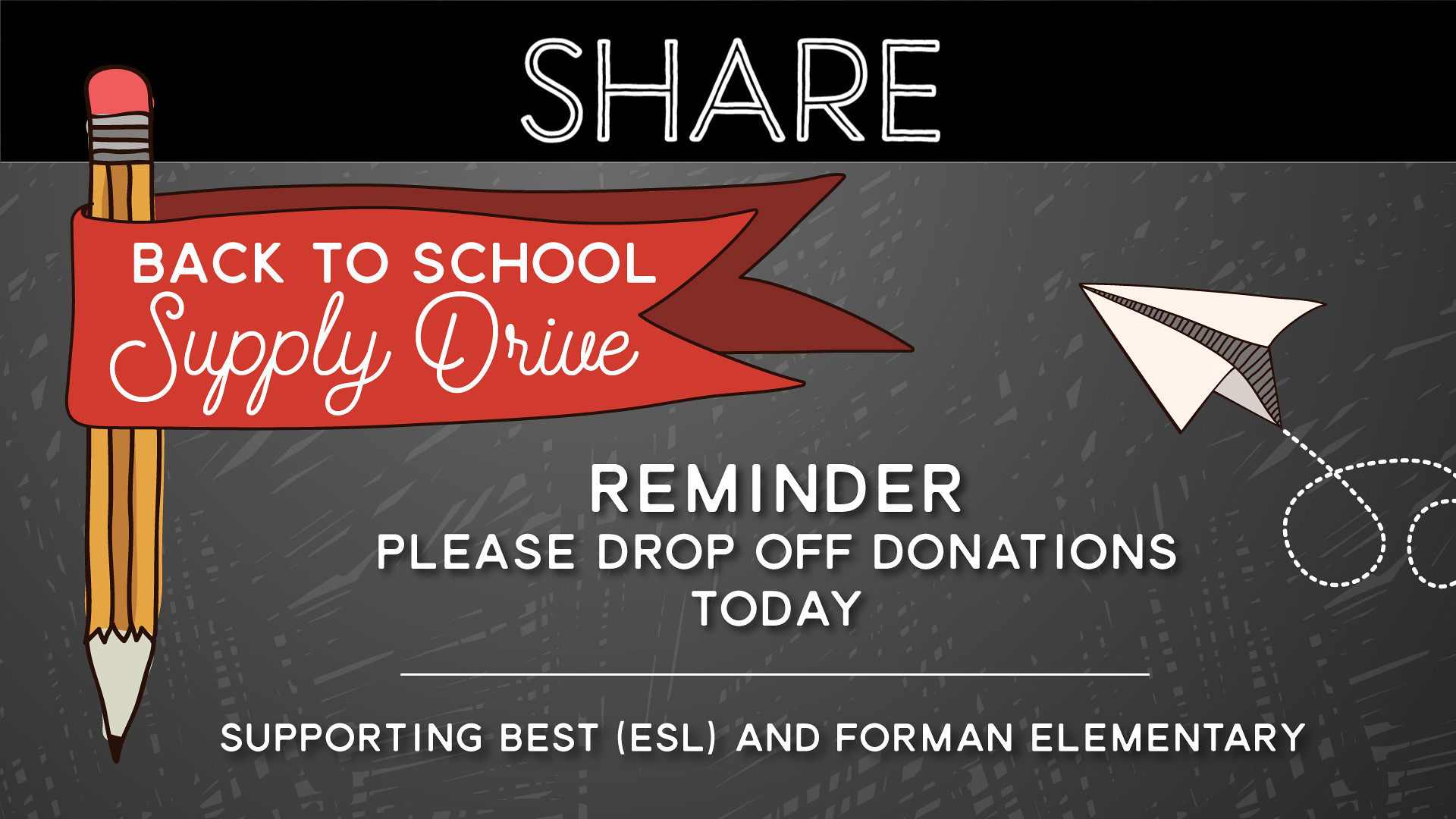The image resembles the size and dimensions of a high-definition television, structured as a rectangular poster. It has a clear school-themed design, dominated by a gray, subtly patterned background interspersed with lines and dashes. At the very top, across a black strip, the word "SHARE" stands out in bold white uppercase letters.

On the left side of the image is a downward-pointing pencil complete with an eraser, detailed with a red banner wrapped around its body. The banner reads "Back to School Supply Drive," with "Supply Drive" elegantly displayed in cursive, setting it apart from the rest of the text. Just to the right of the pencil, there is a playful depiction of a paper airplane, complete with a dotted trail suggesting its flight path, curving and looping through the air.

Centrally positioned in the image is the word "REMINDER," prominently featured in all capital white letters. Directly below, additional instructions read "Please drop off donations today," also in bold white text. A thin white line is placed just beneath this message, serving as a divider. Under this line, the image concludes with the text "Supporting BEST, ESL, and Foreman Elementary," indicating the beneficiaries of the drive.